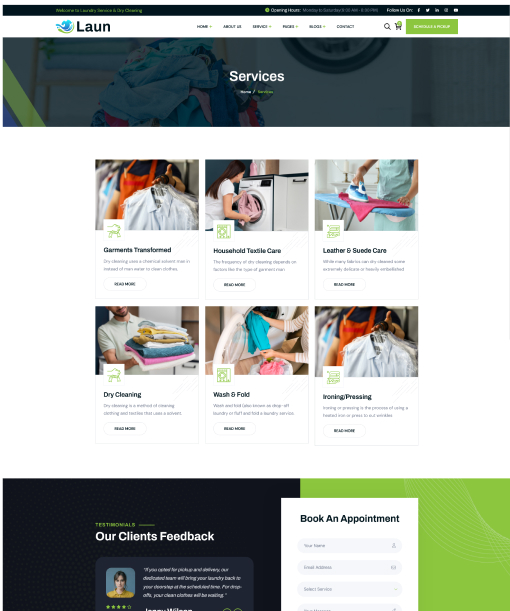The image appears to be a website for a laundry service, titled "LAUN" in the upper left corner. Despite the poor resolution hindering readability of smaller text, the navigation bar includes options such as "Home" with a dropdown menu, a section that seems to start with "Amount," "Services" with a dropdown, another dropdown starting with the letter "P," an unreadable but likely dropdown section, "Contact," a search bar, and a shopping cart icon indicating one item.

Below the navigation bar, a large photograph of a laundromat is partly obscured by a gray overlay with the word "Services" prominently written in white text. Some smaller text in white and green is also present but not legible. 

Further down, there are two rows of three photographs each. The top row includes photos titled "Garment Transformed," "Household Textile Care," and "Leather and Suede Care." The bottom row features "Dry Cleaning," "Wash and Fold," and "Ironing Press." Each section has accompanying descriptive text and a button, both of which are unreadable due to the image resolution.